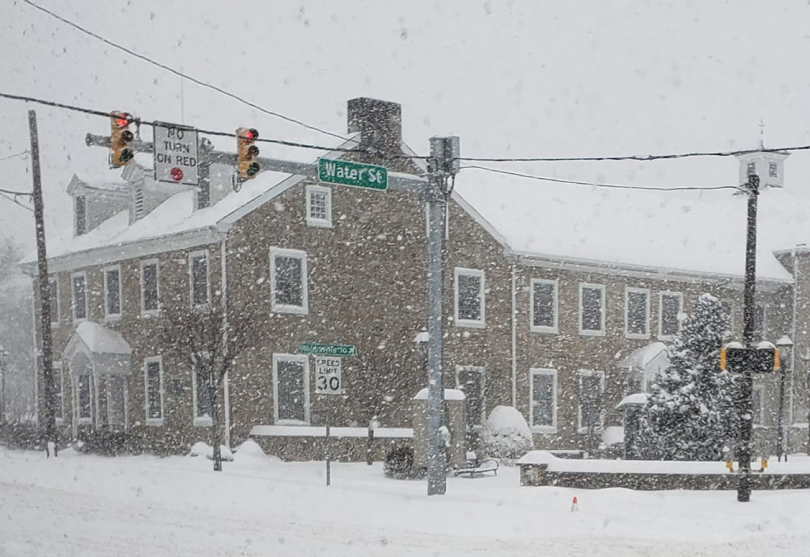This image depicts a bustling intersection in the midst of a heavy snowstorm, where visibility is low due to the snowfall. The primary street, identifiable by a green rectangular sign, is Water Street, intersecting with another street which might be labeled Unionville Square, though the text is obscured. The scene is blanketed in a thick layer of snow, covering the street, sidewalks, trees, and buildings.

Prominently featured are two red stop signs and a silver pole across the intersection, supporting two traffic lights, both glowing red. Below the signals, a white sign with a red circle indicates "No Turn on Red," while a nearby sign denotes a speed limit of 30 mph.

On one side of the intersection stands a large, three-story building with a snow-covered roof and a chimney, its architectural details highlighted by its brown facade and white-framed, tall windows. The structure looms in the background, with snowflakes visibly descending from the sky that mirrors the snowy landscape below, making it difficult to distinguish the horizon. The sidewalk is partially cleared, revealing the snow packed along its edge, adding to the picturesque wintery scene.